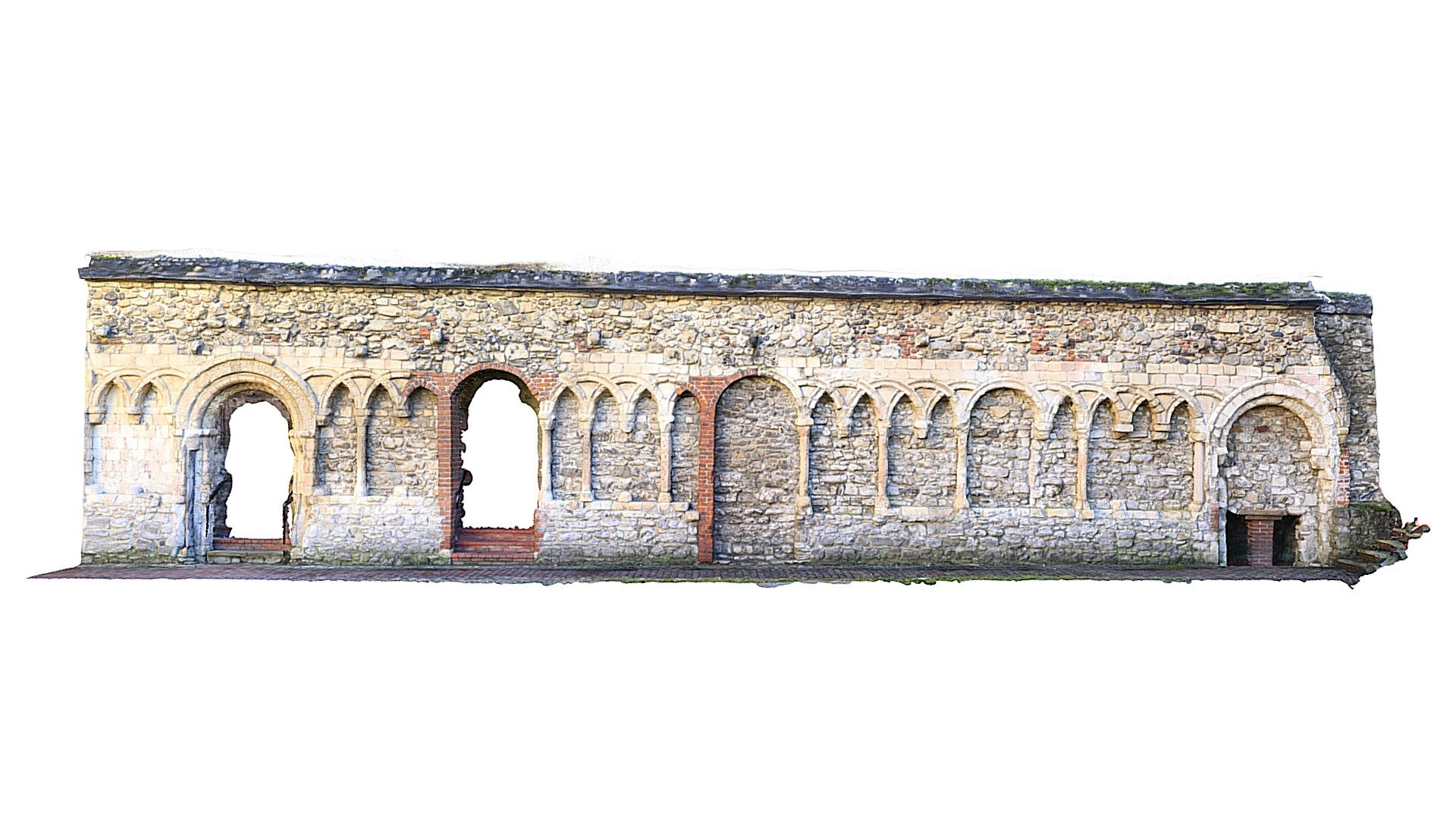The image depicts a preserved section of an ancient wall, which appears to be part of an old building. The wall, constructed from a mix of rock and tan-colored bricks, contains four arched entries. These arches likely served as entrances or exits. The first and second arches have steps leading up to them—two steps for the first and three for the second—indicating they were once functional doors. The third archway is filled with masonry, showcasing the various stone shapes and colors, predominantly white and light brown. There is a unique border design featuring upside-down rings, giving the wall an ornamental touch. At the top of this squat, long wall, a dark charcoal border and a substantial stone section add to its robust yet weathered appearance. The background seems edited out, emphasizing the isolation and preservation efforts for this structure. Despite its age and brittle state, the wall displays signs of meticulous maintenance aimed at safeguarding its historical integrity.